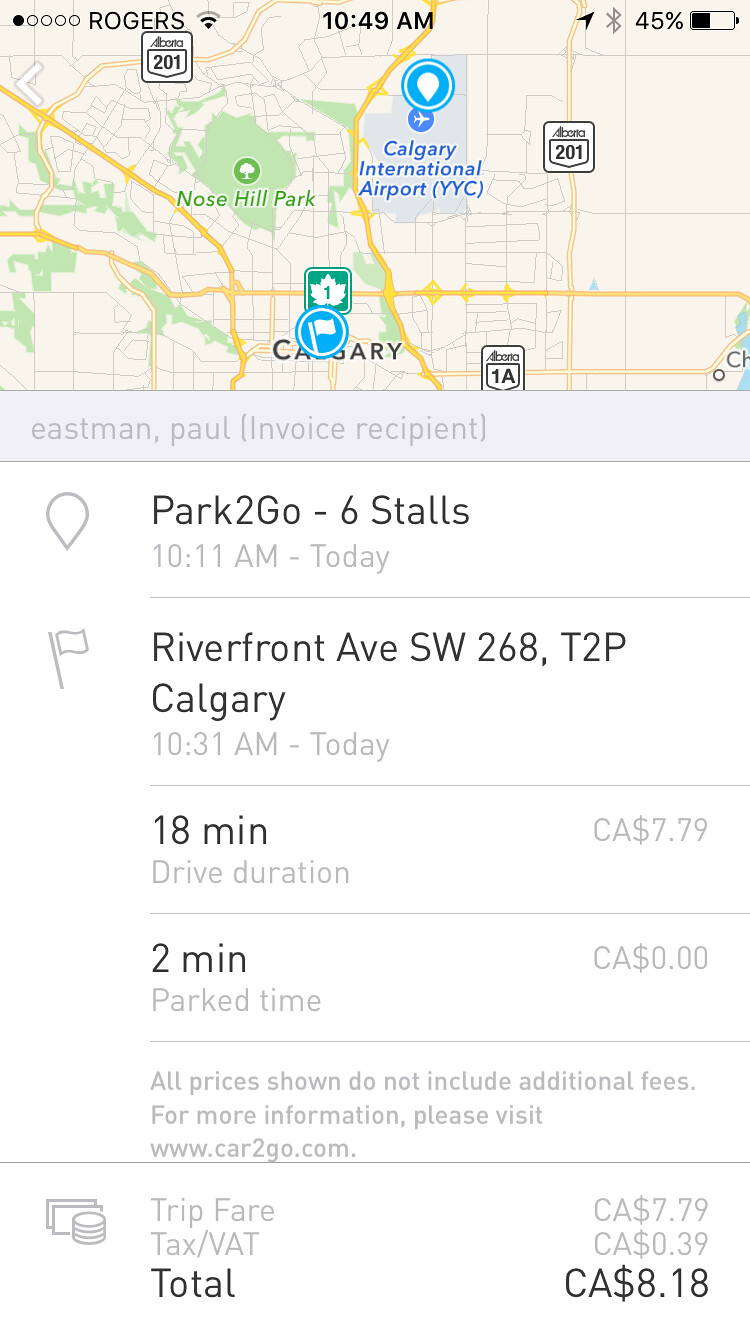This is a screenshot from an iOS device with Rogers as the carrier, taken at 10:49 a.m. The battery is at 45%, with both location services and Bluetooth enabled. At the top, there's a map showing Calgary International Airport (YYC) and the city of Calgary, along with various icons including a leaf, a flag, and three interstate signs for 201 and 1A. This image shows detailed trip information: an invoice receipt for Paul Eastman. The trip starts from Park to Go, which has six stalls available, from 10-11 a.m. today. The destination is Riverfront Avenue SW 268, T2P, Calgary, with an 18-minute drive duration. The cost breakdown includes a trip fare of $7.79 CAD, a tax/VAT of 39 cents, making the total $8.18 CAD. Park time is 2 minutes and free of charge. Additional details mention that prices do not include additional fees and refer users to www.car2go.com for more information.